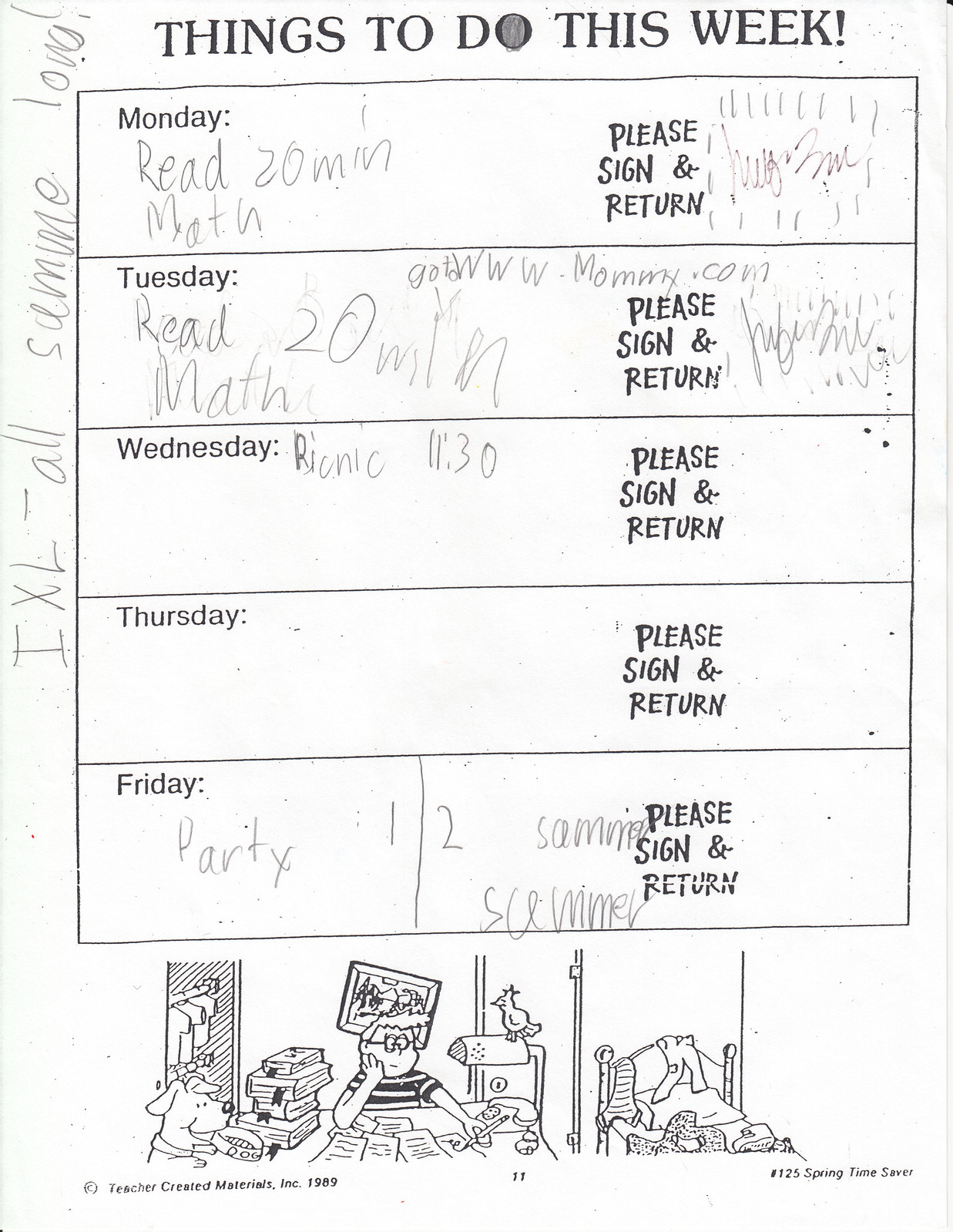This image features a scanned Things to Do This Week sheet that appears to have been filled out by a student. At the very top, in capitalized printed text, it says "Things to Do This Week!" with the student creatively coloring in the 'O' in 'Do.' Down the left side of the sheet, there is a playful note stating "IXL all summer long!" The word 'summer' is misspelled without the 'R', hinting at the student's young age.

The main section of the sheet is divided into a box with days of the week from Monday to Friday. Each day outlines specific tasks:

- **Monday:** Read for 20 minutes and do math. The note "please sign and return" is included, with a parent’s signature and decorative lines drawn around it.
- **Tuesday:** Read for 20 minutes, do math, and visit www.mommy.com. It also has "please sign and return", shows a signature, and has lines drawn around it.
- **Wednesday:** A picnic at 11:30 AM is scheduled, but no signature is present.
- **Thursday:** This section is left blank except for "please sign and return".
- **Friday:** A party is noted, with the words "Sammy", "swimming", and "summer" written.

At the bottom of the page, there is a detailed, cartoonish drawing depicting a busy scene: a boy sits at a cluttered desk with a pencil in his left hand, surrounded by a stack of books, scattered papers, an old-fashioned telephone, and a desk lamp with a bird perched on it. A dog, holding a bowl in its mouth, appears to be asking for food. The background includes a disarrayed bedroom with a bed covered in clothes and shoes, a closet filled with clothes, an open door, and a tilted picture hanging on the wall.